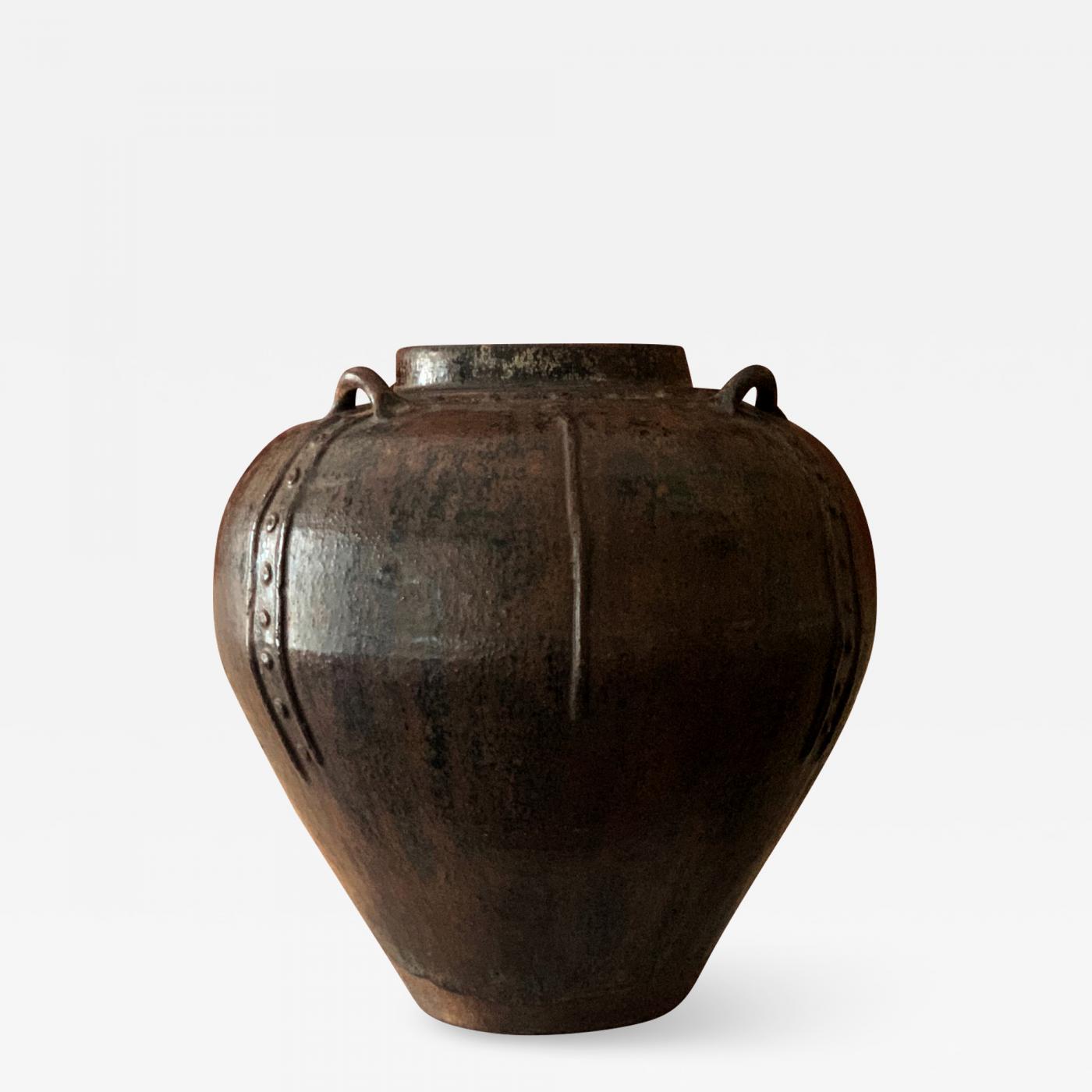The image features a centrally-placed, dark brown urn or piece of pottery with accents of black and possibly copper. The background is predominantly light gray or off-white. The urn, which has an antiquated, rustic vibe reminiscent of Greek or Roman designs, begins with a small, roughly three-quarters-of-an-inch wide base and elegantly broadens outward to form a heart or apple-like shape, albeit with a flat top rather than a pointed or indented bottom. It has a pronounced rectangular lip at the top and two small handles on either side, resembling cat ears. The sides of the urn are adorned with raised vertical stripes, each featuring small raised circles down their centers, giving the piece a beautifully intricate and historic appearance.